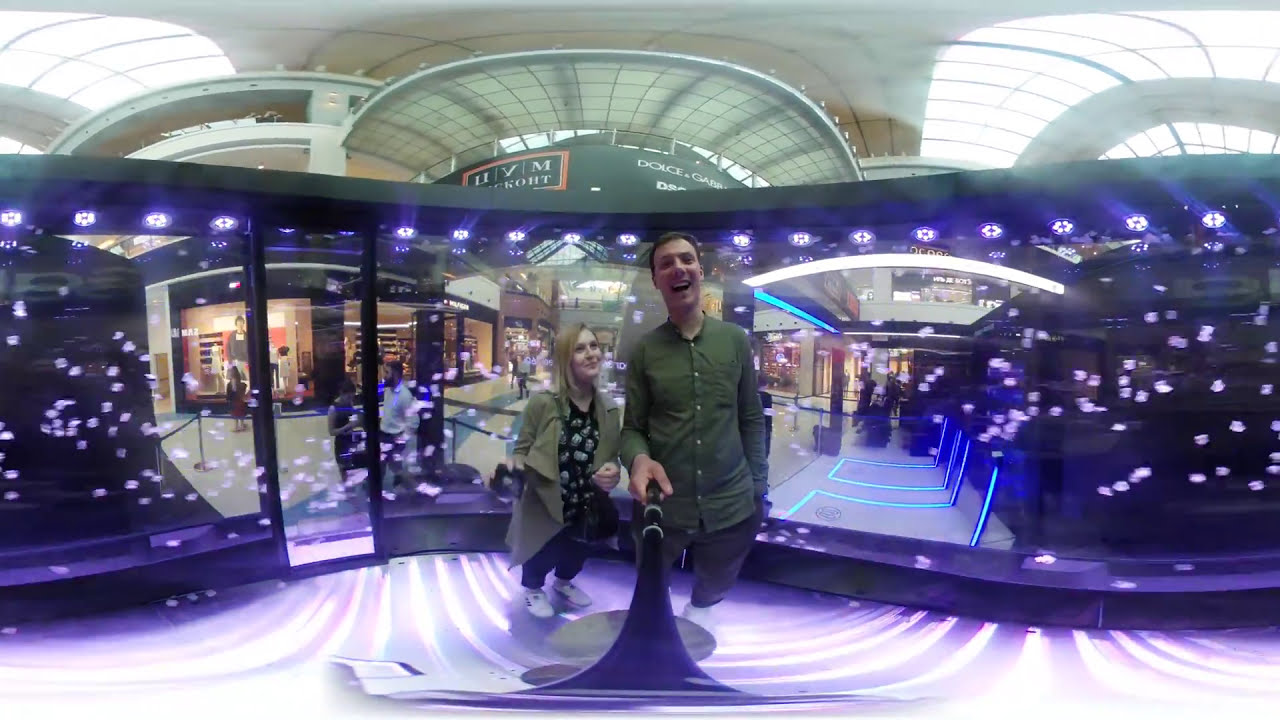A cheerful selfie captures a man and a woman inside a bustling shopping mall. The man on the right, with short brown hair, is holding a black selfie stick with white stripes. He is dressed in a green long-sleeve button-up shirt, dark gray pants, and light white shoes, smiling warmly at the camera. Standing close to him on the left is a woman with blonde hair, wearing a black and white blouse under a long tan trench coat, black pants, and white sneakers. Their backdrop is a striking glass display adorned with purple LED lights, creating an eye-catching frame. Floating objects, resembling money, can be seen swirling within the display, contributing to the futuristic ambiance. Behind this unique installation, store signs, including Dolce & Gabbana, indicate the lively mall setting with multiple shops and people bustling around. The scene is slightly distorted, adding a dynamic feel to the photo.